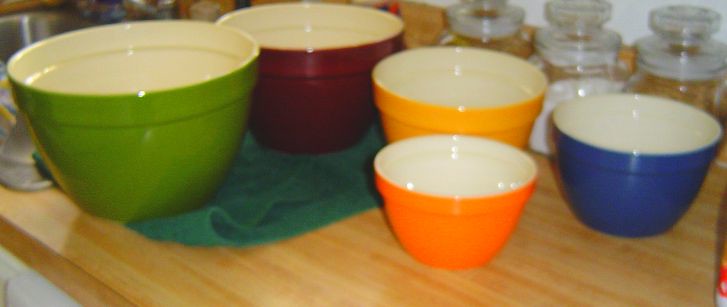This image features a meticulously arranged set of five colorful ceramic bowls placed on a light wooden kitchen countertop. Each bowl is white on the inside but sports a vibrant exterior color: the largest bowl on the far left is green, followed by a slightly smaller red bowl. Both of these bowls rest on a green towel. To the right of these are progressively smaller bowls - a yellow one, then a blue one, and finally, the smallest bowl is orange. In the background, behind these bowls, are three empty, see-through glass jars. The entire setup is positioned next to a kitchen sink, which can be seen in the background. The detailed arrangement and variety of colors create a visually appealing scene of kitchenware.